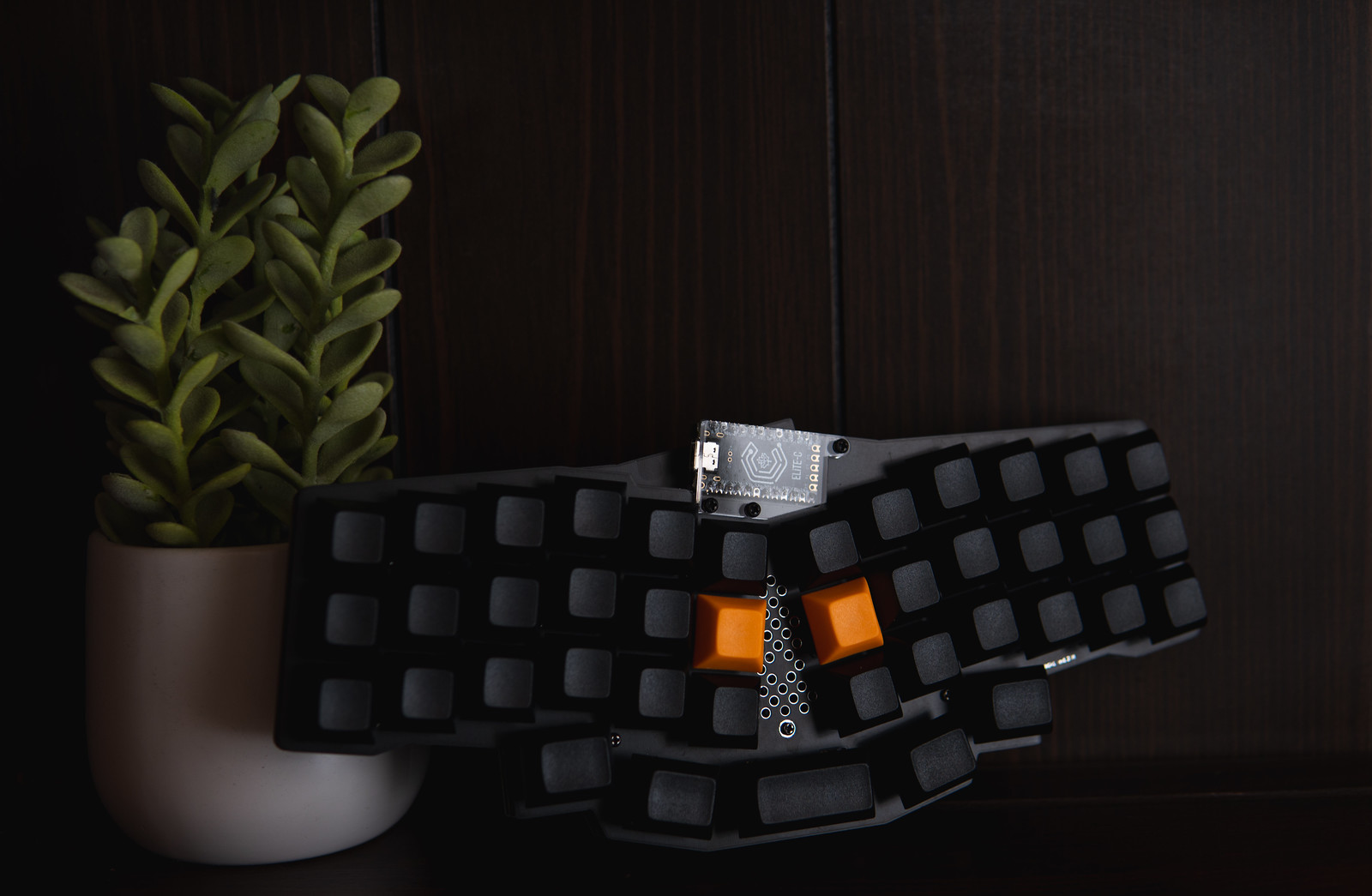The image depicts what appears to be a uniquely designed keyboard laid against a dark brown wooden table. The keyboard is split into a V-shape, with each side featuring multiple rows of small, raised black keys that lack any visible text. At the center of this split keyboard are two orange keys, one on each side, with a small flat ridge between them. The keyboard, constructed from black plastic, has a solid black background. 

Behind the keyboard, there's a purple pot housing a green plant with three visible stalks, each adorned with numerous leaves. Additionally, off to the left side of the image, a short gray vase contains light green stalks with small, matching green leaves.